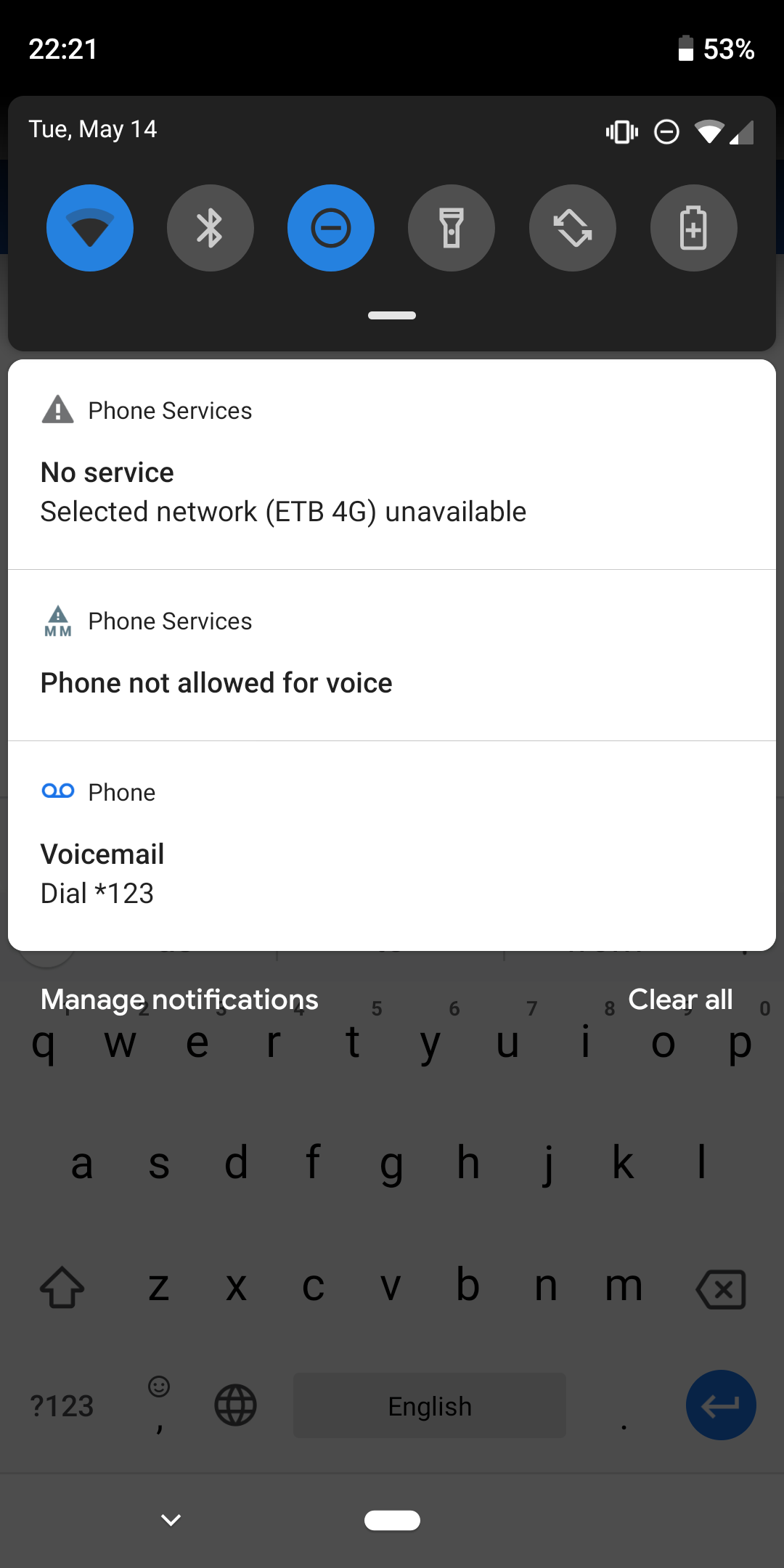A detailed screenshot displays a mobile phone interface. At the top, a darker black banner contrasts with a black background, showcasing the time on the left in 24-hour format (22:21) and the battery level at 53% on the right. Below this, a slightly lighter grey rectangular bar indicates the date, Tuesday, May 14th. Various icons for network status, Wi-Fi, Bluetooth, and other settings are visible adjacent to the date.

Beneath this grey bar, a notification panel lists three alerts. The first two notifications are related to phone services: the initial message reads, "No service. Selected network unavailable," and the second states, "Phone not allowed for voice." The third notification, from voicemail, instructs the user to "Dial 123 to access voicemail."

The background reveals the device’s QWERTY keyboard, which appears grayed out and subdued due to the active notification panel overlaying it.